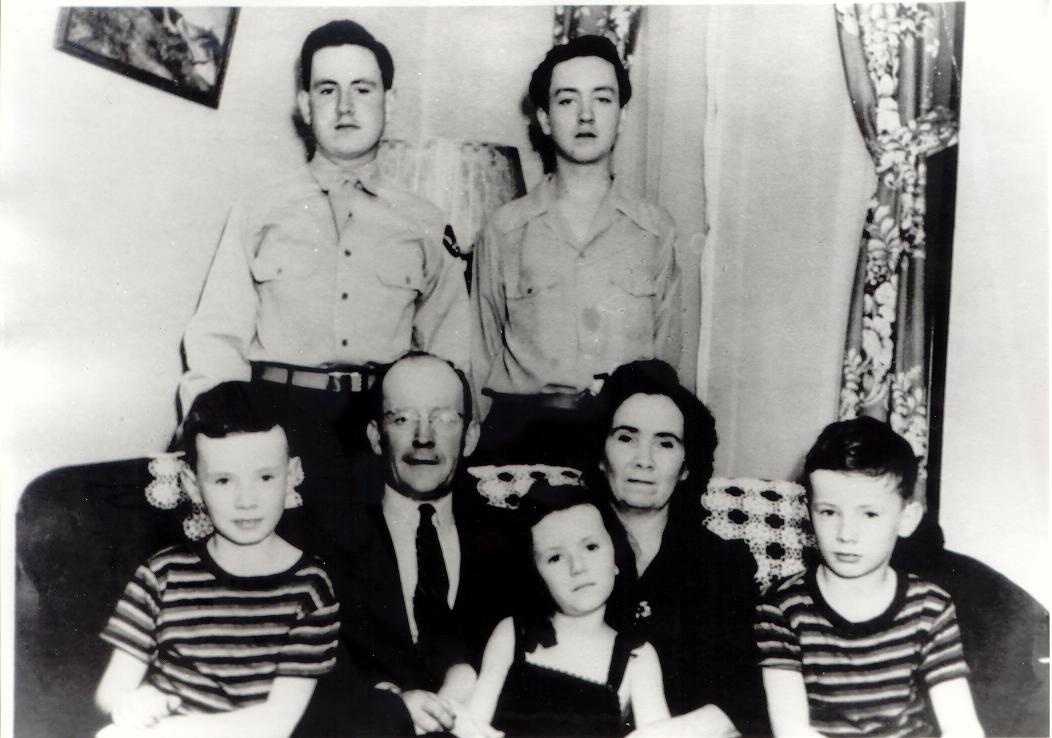The photograph is a highly detailed, black-and-white image of a family composed of seven members. Seated on a dark-colored couch at the forefront are an elderly man and woman flanked by three children. The younger boys, who appear to be in elementary school, are wearing short-sleeved black and white t-shirts, while a little girl at the front is dressed in a black tank shirt. Standing behind the couch are two older boys, likely the teenagers of the family, dressed in long-sleeved, collared button-down shirts. The scene is set inside their home, as evidenced by a window with curtains and a picture frame mounted on the wall to the left. Despite the serious expressions on their faces, the photograph is notable for its clarity and the stark contrasts of black, white, and shades of gray, giving it a timeless quality.